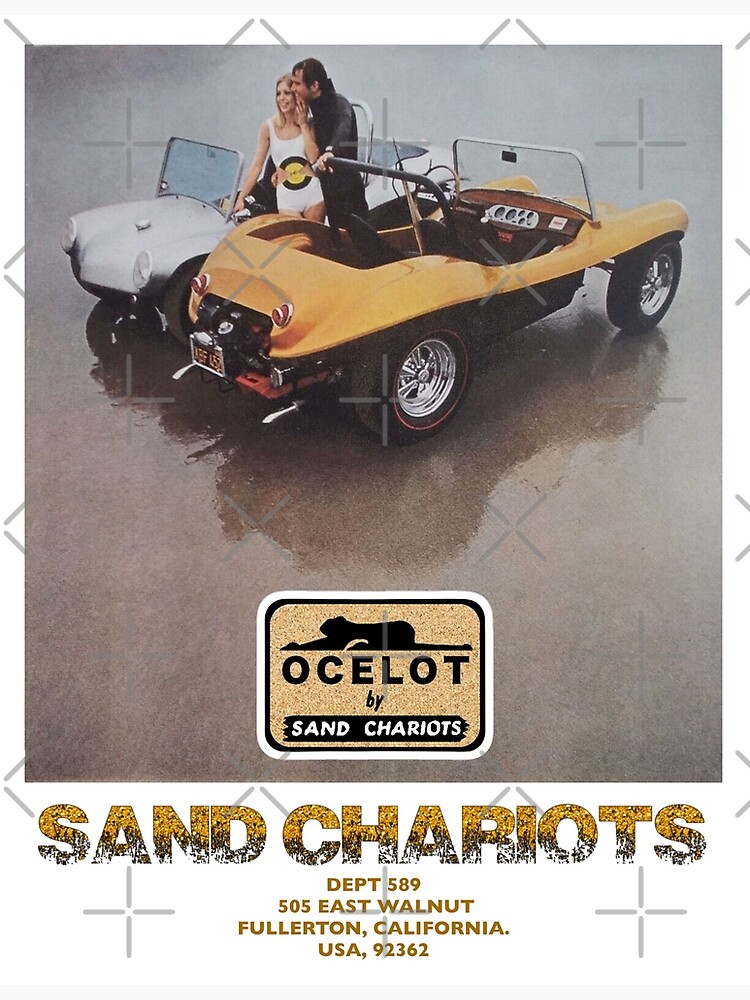The image appears to be a vintage advertisement from the late 60s or early 70s showcasing two dune buggies. In the center, just in front of the vehicles, stands a couple likely in their 30s. The woman is on the left, dressed in a white swimsuit adorned with a circle featuring a black edge and a yellow center on her belly. The man, standing to the right, wears a black outfit. Both cars are roofless convertibles; the car on the left is white, and the one on the right is yellow, though one caption mentions it might appear more orange. The scene is set on a hard, shiny floor rather than sand. Below the image is a rectangular logo that reads "OZELOT by Sand Chariots." Beneath the logo, in an orangish-yellow font against a white background, the text reads "Sand Chariots, Department 589-505 East Walnut, Fullerton, California, USA, 92362."